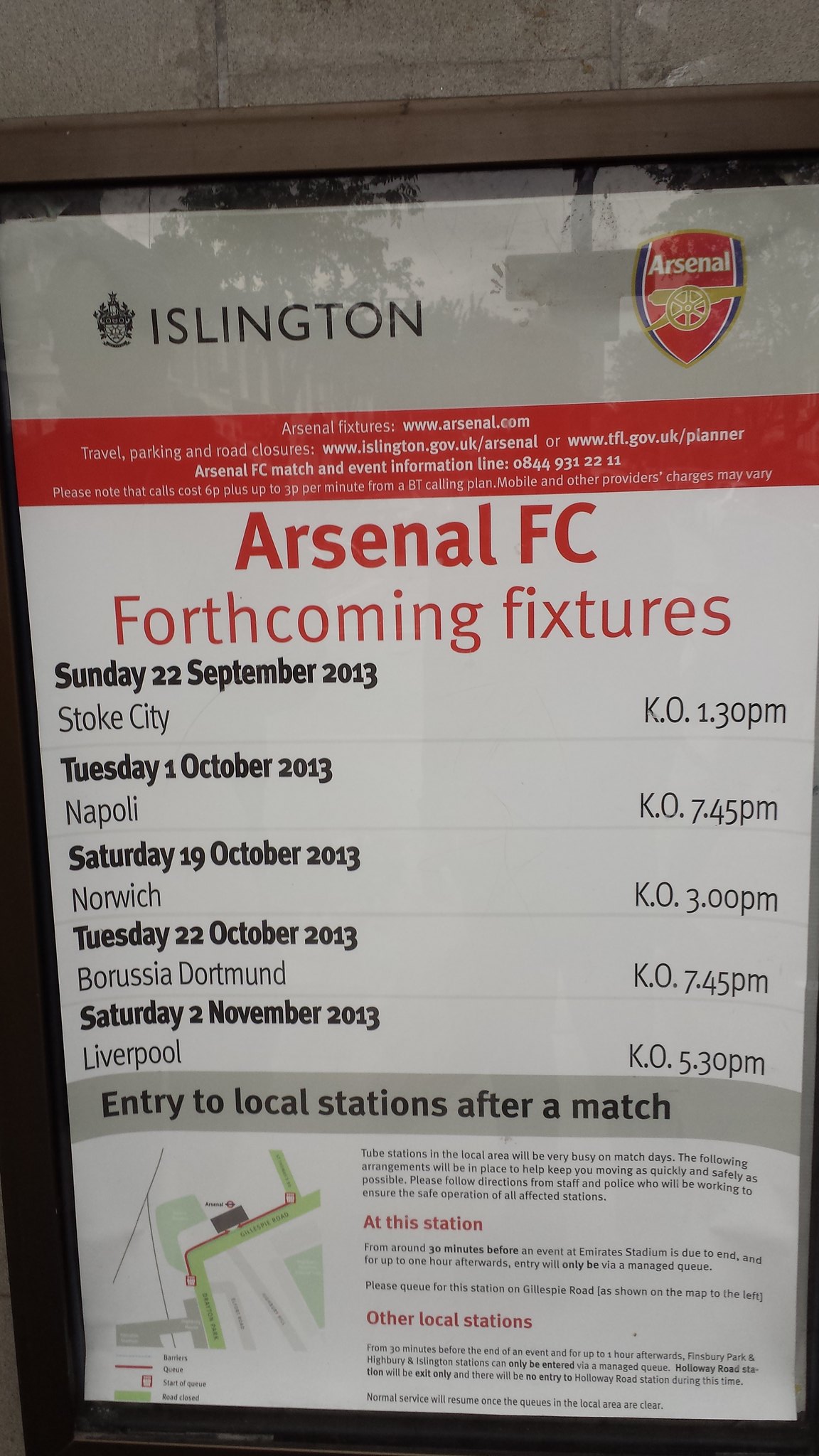The image features a centrally positioned sign, possibly viewed through glass, suggesting it might be against a building or inside a store window, likely outdoors in the middle of the day. The sign is on a long, white paper with a schedule of Arsenal FC's forthcoming fixtures prominently displayed. At the top, the sign reads "Islington" in black, with a red shield featuring a gold-colored cannon on a wheel to the right. Below, the sign prominently states "Arsenal FC Forthcoming Fixtures" in large red letters. The schedule lists several dates: Sunday 22 September 2013 against Stoke City (K.O. 1.30 p.m.), Tuesday 1 October 2013 against Napoli (K.O. 7.45 p.m.), Saturday 19 October 2013 against Norwich, Tuesday 22 October 2013 against Borussia Dortmund, and Saturday 2 November 2013 against Liverpool. The bottom section includes information about entry to local stations after a match, accompanied by a map and additional text. The diverse color scheme includes white, black, tan, green, gray, red, yellow, gold, and light blue.